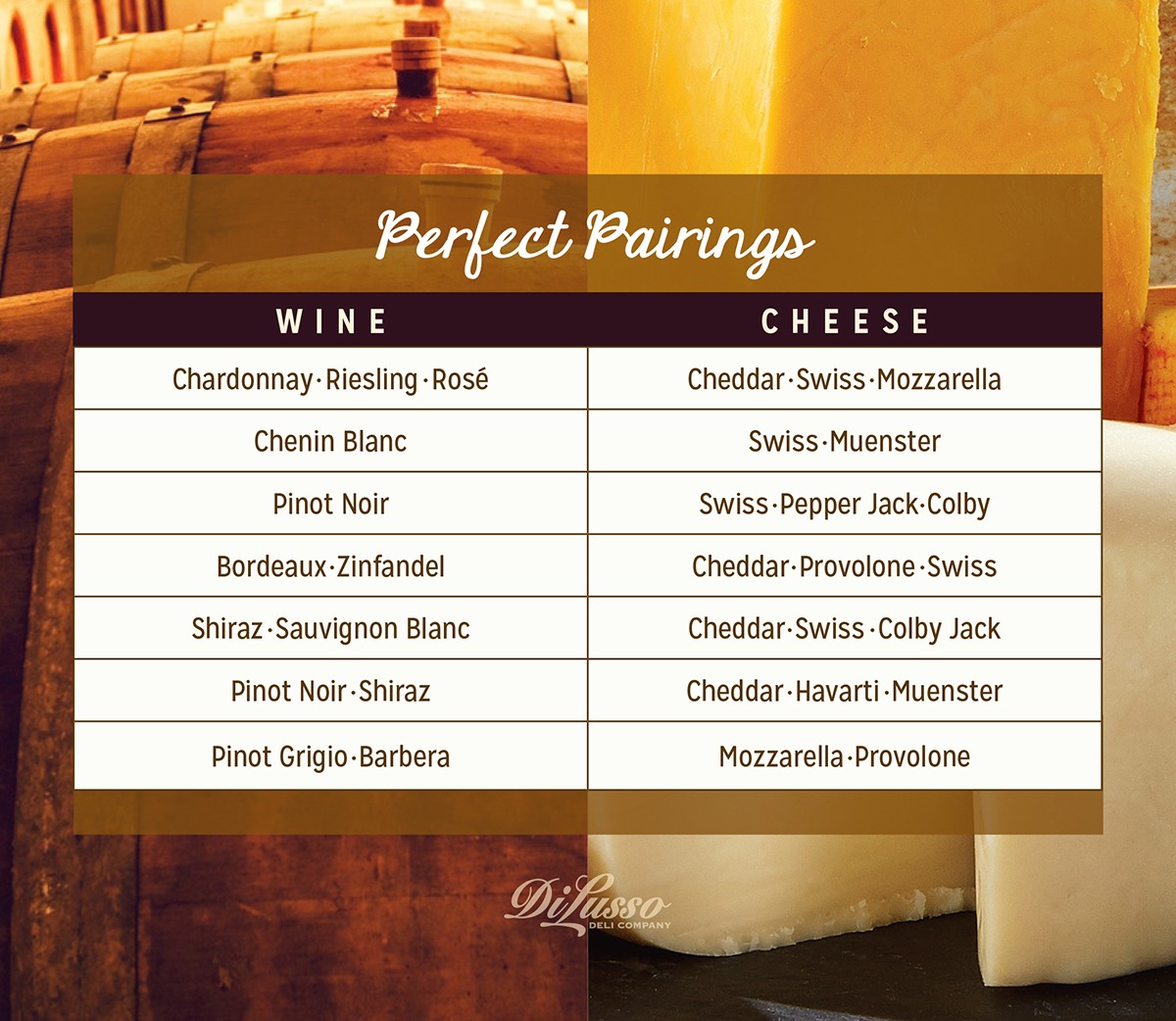The image, titled "Perfect Pairings," is a chart depicting ideal wine and cheese combinations. The chart consists of two columns with the left labeled "Wine" and the right labeled "Cheese," featuring seven pairings. The listed pairings are as follows: Chardonnay, Riesling, and Rosé with Cheddar, Swiss, and Mozzarella; Chenin Blanc with Swiss and Munster; Pinot Noir with Swiss, Pepper Jack, and Colby; Bordeaux and Zinfandel with Cheddar, Provolone, and Swiss; Shiraz and Sauvignon Blanc with Cheddar, Swiss, and Colby Jack; Pinot Noir and Shiraz with Cheddar, Havarti, and Munster; and Pinot Grigio and Barbera with Mozzarella and Provolone. The background showcases two photos: wooden wine barrels on the left and blocks of cheese on the right. The bottom center of the image displays the name "DeLusso Deli Company."